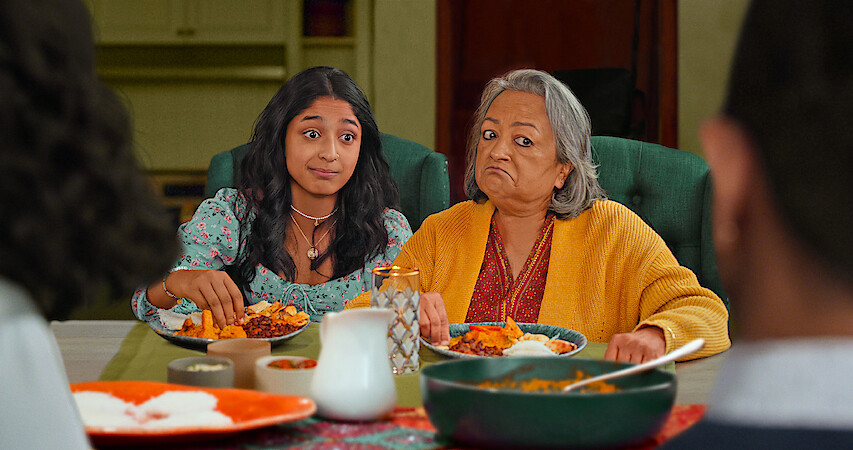The photograph depicts an intimate and possibly tense moment between an older woman and a young girl, seated at a table and facing two other individuals whose faces are turned away from the camera. The older woman, positioned on the right, wears a yellow sweater over a red v-neck top adorned with floral patterns. Her short, whitish hair frames a skeptical expression as she scrutinizes the scene before her. In front of her is a plate containing what appears to be tacos with salsa and sour cream. 

The younger girl, situated on the left, has long, curly dark hair and dark skin, suggesting she might be of Indian descent. She wears a distinctive choker necklace with a gold charm and a blue, flower-patterned top. Her expression, featuring raised eyebrows and a closed mouth, conveys a mix of curiosity and bemusement as she looks towards the two obscured figures. Her hands are in her food, which looks similar to the older woman's meal, possibly consisting of beans or curry chicken on a colorful plate.

The table is adorned with several items: small containers of dip, a white creamer, a glass with white and green patterns, and a green bowl with a large spoon. They are seated on high-backed green armchairs, with greenish placemats used for the setting. The background reveals a lime green backboard, cupboards, white shelves, and part of a doorway, all lending to a green and brown kitchen motif. An orange plate and a candle with gold emblems add additional color and detail to the scene.